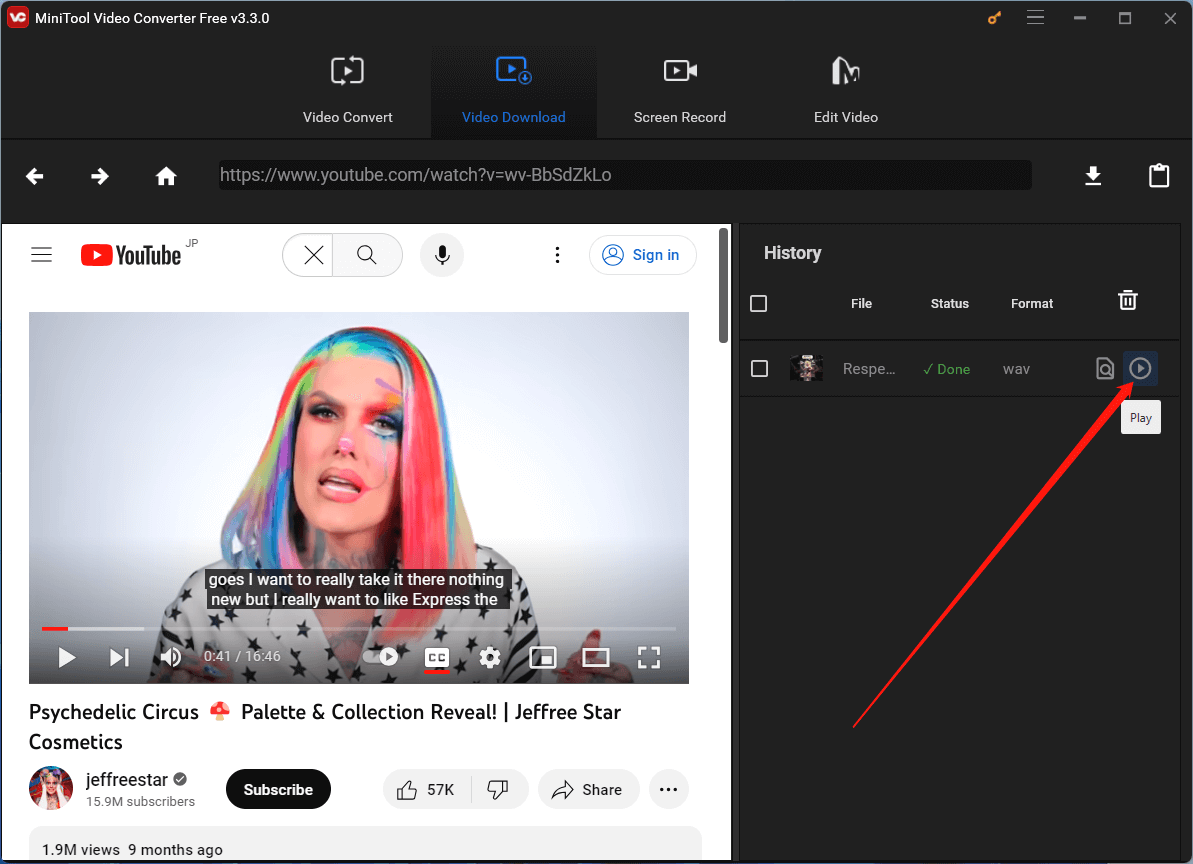This image is a detailed screenshot showcasing a user interface of the MiniTool Video Converter (free v3.3.0). It prominently features a YouTube video being converted within this software. The top left corner displays the MiniTool logo: white "BC" letters inside a red, rounded square, accompanied by the software version. The overall user interface is a dark theme, primarily black or dark gray. 

In the top right corner, various icons are visible: a yellow key, a hamburger menu, a minimize button, a maximize/restore button, and a close (X) button. The central part of the interface contains four main tabs: "Video Convert," "Video Download," "Screen Record," and "Edit Video." The "Video Download" tab is selected, indicated by its black background and blue text and icon.

Below the tabs, there is a mini browser interface with back, forward, and home buttons in white. The URL field contains a YouTube link: "watch?v=WV-BBSDZKLO," and next to it are a download button and a clipboard icon. Under this section is a preview window of the YouTube video, which features the title "Psychedelic Circus with Mushroom Icon Palette and Collection Reveal | Jeffree Star Cosmetics." The paused video shows Jeffree Star speaking against a light gray background.

The video information displayed includes Jeffree Star's channel with 15.9 million subscribers, 57,000 likes, a dislike button, a share button, a three-dot menu, 1.9 million views, and the video upload date of nine months ago. 

To the right of the video preview, there is a "History" section with columns titled: Checkbox, File, Status, Format, and a Delete icon. A row in this section shows the file named "REAPE..." with a status of "Done" in green, format "WAV," and has a play icon. This play icon is specifically highlighted with a red arrow added by the user for emphasis.